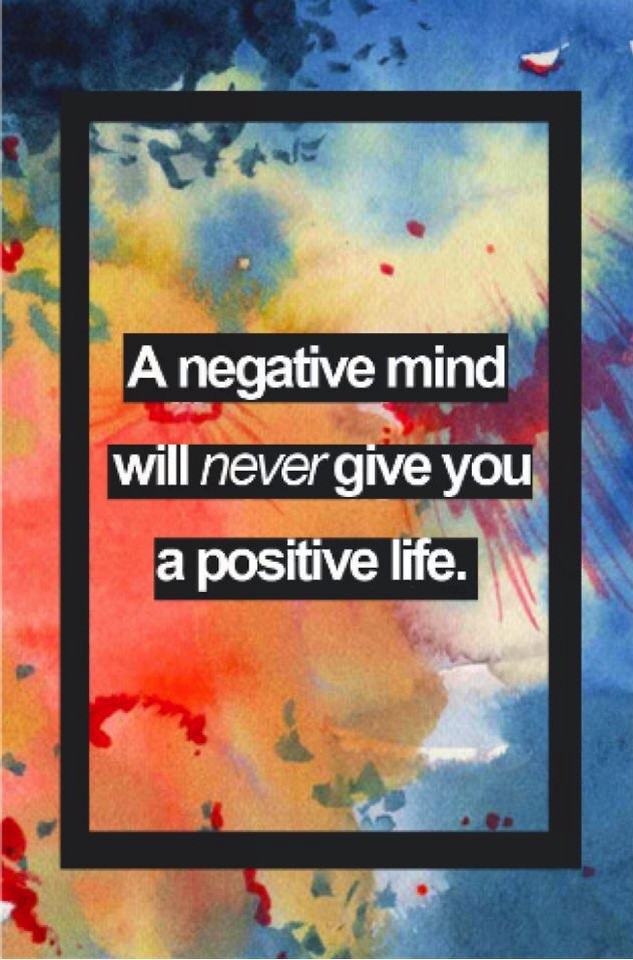A vibrant sign against a black background features the motivational quote: "A negative mind will never give you a positive life." The text is elegantly rendered in white lettering, enclosed within a black square frame. Multicolored accents adorn the sign, enhancing its visual appeal and emphasizing the uplifting message.